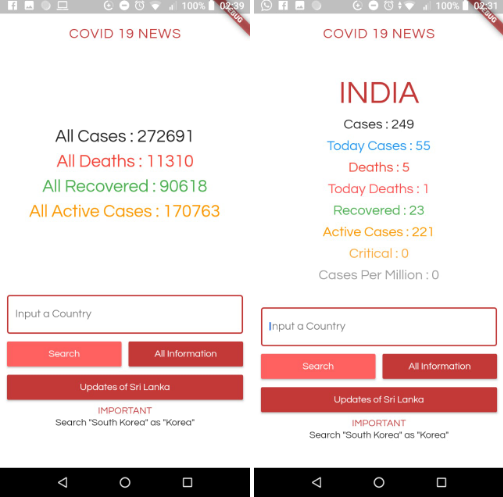This image showcases a screenshot taken from a mobile app, and it features two side-by-side panels. Both panels have a similar layout but display different COVID-19 statistics.

On the left panel, titled "COVID-19 News," the data highlights global statistics:
- Total cases: 272,691
- Total deaths: 11,310
- Total recovered: 90,618
- Total active cases: 170,763

Below these figures, there are options to input a specific country, a search function, and an informational key.

The right panel displays COVID-19 statistics specifically for India, with the title "India" prominently highlighted in red. The data includes:
- Total cases: 249
- Today's cases: 55
- Total deaths: 5
- Today's deaths: 1
- Total recovered: 23
- Total active cases: 221
- Critical cases: 0
- Cases per million: 0

Similar to the left panel, the bottom section of the right panel provides options to input a country, search, and access all relevant information.

Both images have a unified design, emphasizing their related but distinct content.